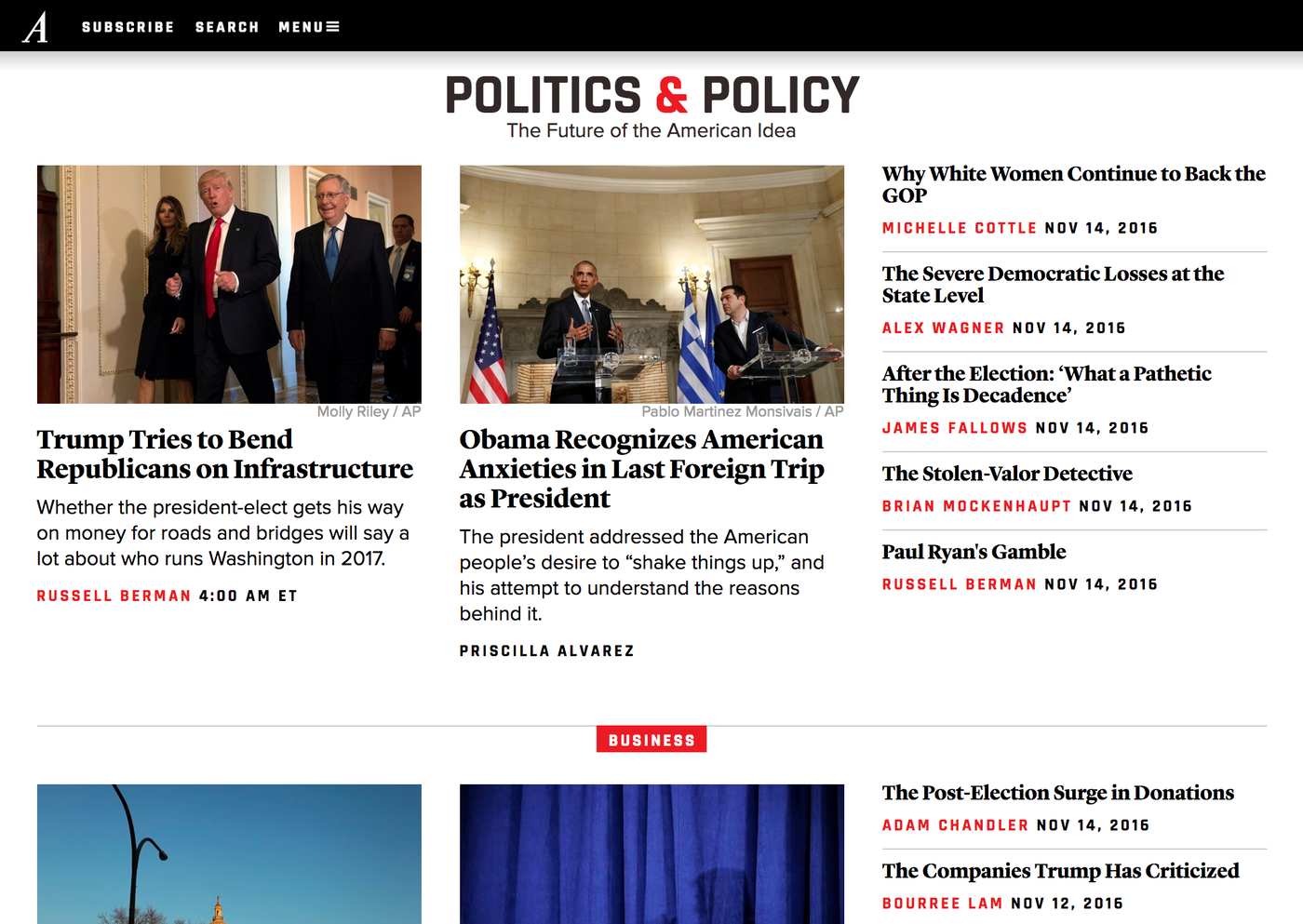The image displays a collage of various news articles. At the top, a black bar contains options for "Subscribe," "Search," and "Menu" in white text. Below this, the main header spells "POLITICS & POLICY" in bold uppercase black letters, with the ampersand in red. 

Beneath the header is a subheading reading "The Future of the American Idea" in black lettering. The primary visual element features a photograph of Donald Trump wearing a black suit and a red tie, flanked by two other individuals. Below this image, a caption in black text reads "Trump Tries to Bend Republicans on Infrastructure," with the article authored by Russell Berman, noted in red text, and time-stamped at 4 a.m. Eastern-time.

To the right, there is another image showing Barack Obama at a podium, with another man at a separate podium looking towards him. The caption underneath reads, "Obama Recognizes American Anxieties in Last Foreign Trip as President" in black text.

Additionally, a small red rectangle with white text states "Business." Adjacent to this, black text reads, "Why White Women Continue to Back the GOP."